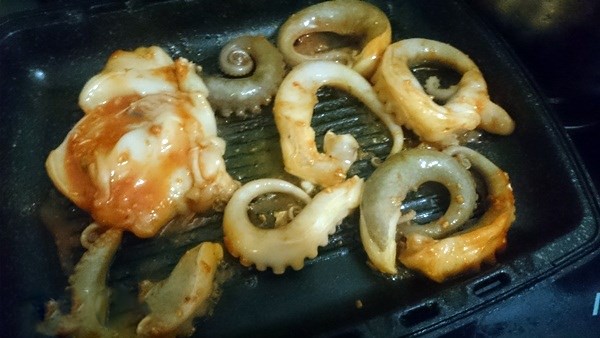The photograph depicts a close-up of an indoor black metal grill with large ribbed squares, set on a blue cloth. Arrayed on the grill are meticulously chopped pieces of what appear to be octopus arms, showcasing their distinctive white ridges and tentacle shapes. These arms, eight in total, are scattered primarily toward the right and bottom left sections of the grill. Their glistening, wet, and slightly slimy texture reflects hues of white and gray. In the top left corner of the grill rests a larger chunk of meat, presumed to be the body of the octopus. This main part is characterized by its pink and white coloring, suggesting a layer of fat and a hint of blood, with a notable red section. The dark background accentuates the vivid details of the seafood, ready to be cooked for an upcoming meal.